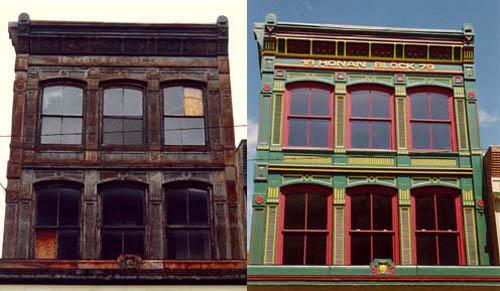The image features two side-by-side photographs depicting a transformative renovation of a two-story, arched-window building. The left photograph shows the "before" state, where the structure appears extremely weathered, rusted, and dirty. The paint is dark brown, and there are six large windows—three on each floor—with noticeable damage: panes are missing and replaced by plywood in the upper right and bottom left corners. Despite its dilapidated condition, the building’s robust framework remains evident.

In stark contrast, the right photograph captures the building on a sunny day with a blue sky, revealing its full refurbishment. The building has been beautifully repainted in green with ornate yellow and red trim. The window frames are now a vibrant red and all the windows are arched and pristine. The text on the building, painted in yellow, reads "Honan Block 29." The restoration also highlights architectural details, enhancing the building's historical charm with its newly vibrant colors and restored structure.